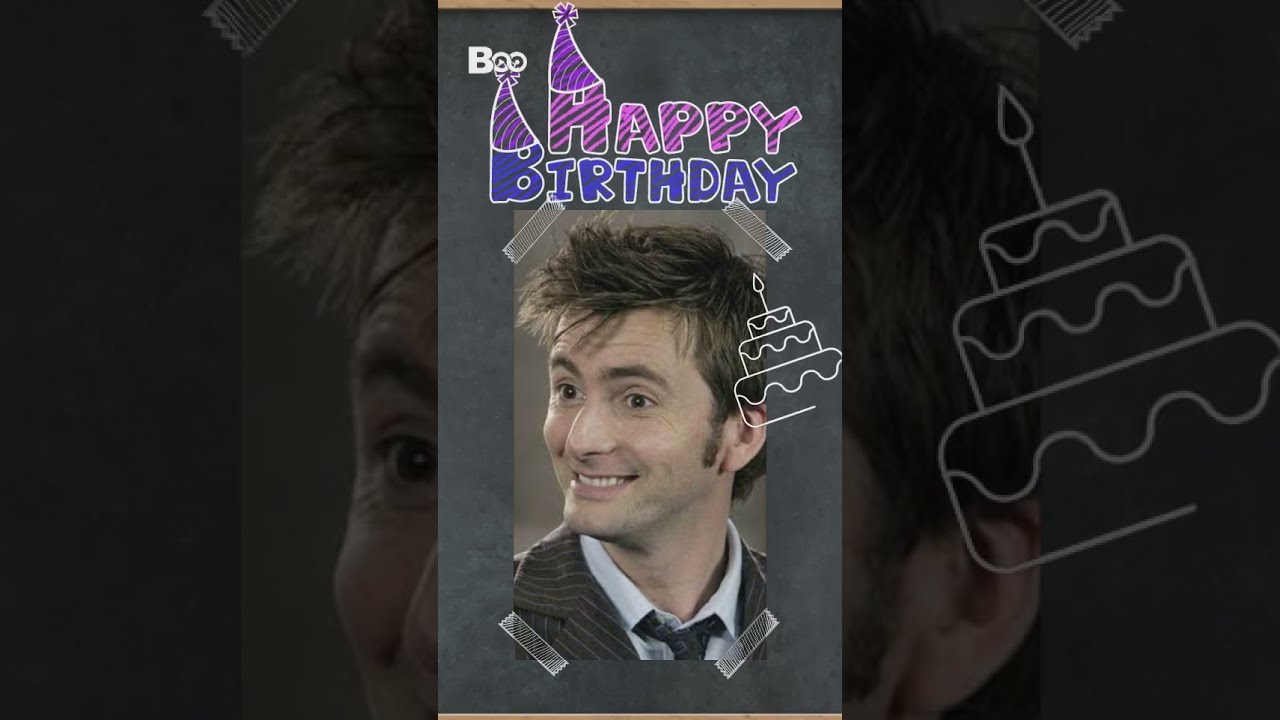The image showcases a creatively designed digital birthday card featuring David Tennant as the 10th Doctor Who. In the center, a photograph captures Tennant with his signature messy hair, expressive raised eyebrows, and a charming, slightly cheesy grin. He is dressed in a pinstripe gray suit jacket over a white button-up collared shirt and a gray tie. His face, with fair skin and brown eyes accented by a faint stubble, looks off to the left-hand side.

The photo appears to be taped onto a gray paper background, mimicking a blackboard, and above it, the word "BOO" is written in white print. Below, "HAPPY" is spelled out in a playful purple hue with pink stripes, adorned with a purple and pink birthday hat perched on the H. The next line features the word "BIRTHDAY" in purple with a white outline, and a similar hat decorates the B. Overlapping Tennant’s left ear is a white line drawing of a three-tiered birthday cake with a candle on top.

In the background, a blown-up, darkened version of Tennant’s face stretches across the layout, with an enlarged view of his left ear and the birthday cake drawing. This creates a layered effect, emphasizing the celebration theme with repeated elements and bold, vibrant text that looks as if it were written with chalk on a blackboard. The card artfully combines whimsy and fandom, making for an engaging and dynamic birthday greeting.